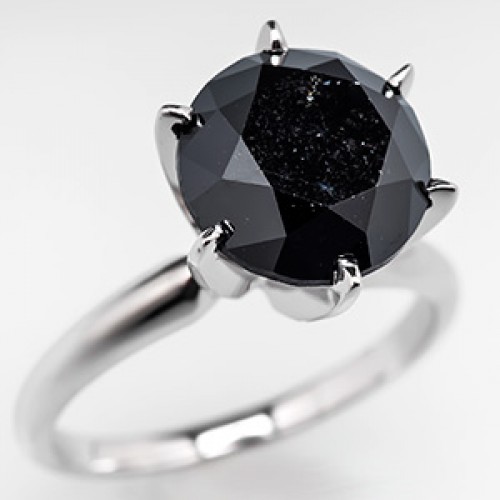In this close-up image, a striking ring is showcased against a pristine white background. The ring features a circular-cut stone, which appears to be a black onyx, set in a simple yet elegant round silver band. The stone is securely held in place by six silver clasps. Light reflecting off the ring creates a captivating effect, enhancing the contrast between the dark onyx stone and its subtle white markings. The top of the stone appears particularly dark, amplifying the intricate reflections and details. The silver band appears slightly blurred, emphasizing the focus on the stunning stone and its meticulous setting.